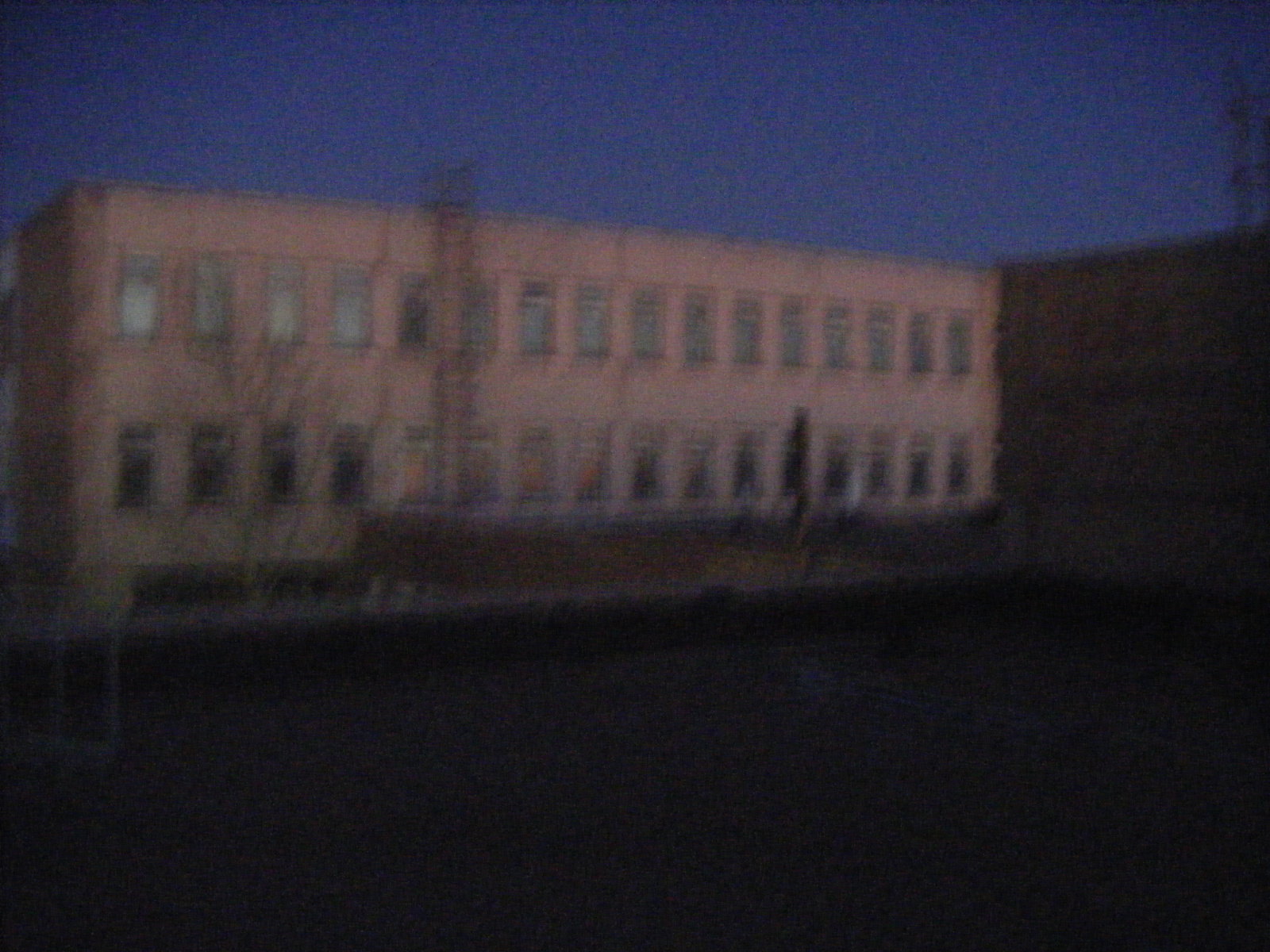In this night-time image, the scene is notably blurry, capturing a view from an elevated vantage point, possibly a balcony. The dark blue sky forms the backdrop, adding to the nocturnal ambiance. Dominating the foreground is a dimly visible wall, hinting at the balcony's structure. Beyond this, a red brick building stands prominently, distinguished by multiple windows, suggesting it could be an apartment building or a school. On the right side, there's a vague outline of another structure, which could either be part of the same building from which the photo was taken or a separate adjacent building. Attached to the side of the red brick building is an indeterminate object, possibly construction scaffolding or a ladder, adding an element of intrigue to the scene.